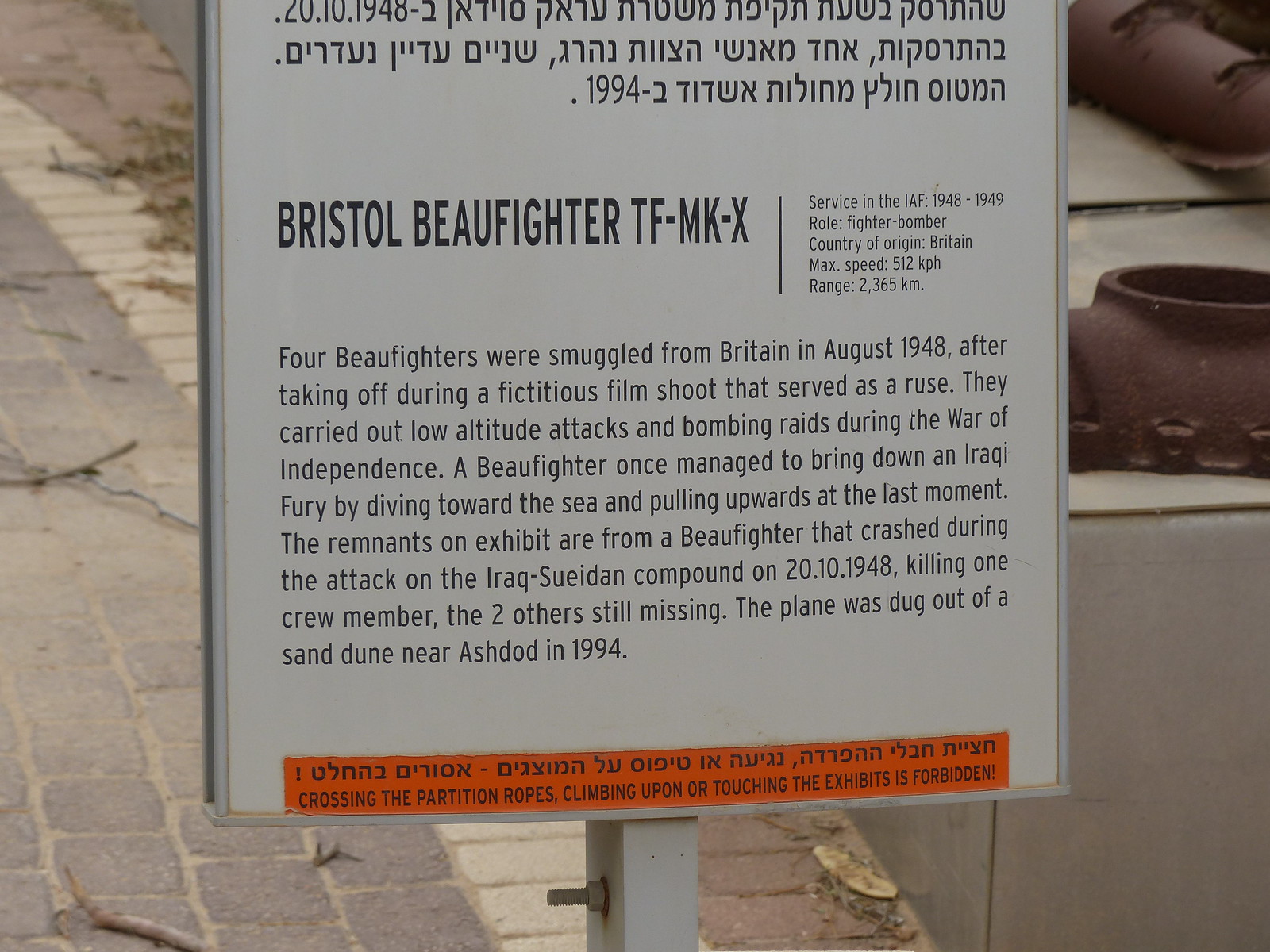The image depicts a close-up of an informational sign mounted on a white metal post secured with a bolt. The sign, bordered by silver metal, stands over a stone walkway, with some indistinct metal objects visible to the right. The uppermost part of the sign possibly contains characters from a non-Latin script, which might be Arabic. Below this, prominently in bold black letters, it reads "Bristol Bowfighter TF-MK-X."

The accompanying paragraph explains that four Bowfighters were smuggled from Britain in August 1948 under the guise of a film shoot. These aircraft carried out low-altitude attacks and bombing raids during the War of Independence. One notable Bowfighter successfully brought down an Iraqi Fury by diving toward the sea and pulling up sharply just in time. The remnants displayed are from a Bowfighter that crashed during an attack on the Iraq-Syrian compound on October 20, 1948, resulting in the death of one crew member, with two others still missing. The wreckage was eventually excavated from a sand dune near Ashdod in 1994.